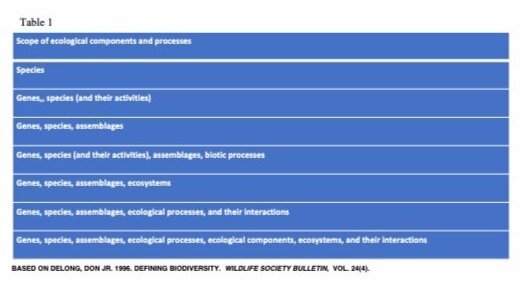**Table 1: Scope of Ecological Components and Processes**

*This table exemplifies the various scopes of biodiversity as defined by different sets of ecological components and processes. Derived from DeLong, Don Jr. (1996), Wildlife Society Bulletin, Volume 24(4).*

| **Ecological Components and Processes** |
|-----------------------------------------|
| Genes, species, and their activities     |
| Genes, species, assemblages              |
| Genes, species, and their activities, assemblages, biotic processes  |
| Genes, species, assemblages, ecosystems  |
| Genes, species, assemblages, ecological processes, and their interactions |
| Genes, species, assemblages, ecological processes, ecological components, ecosystems, and their interactions |

*Based on DeLong, Don Jr. (1996). Defining biodiversity. Wildlife Society Bulletin, Volume 24(4).*